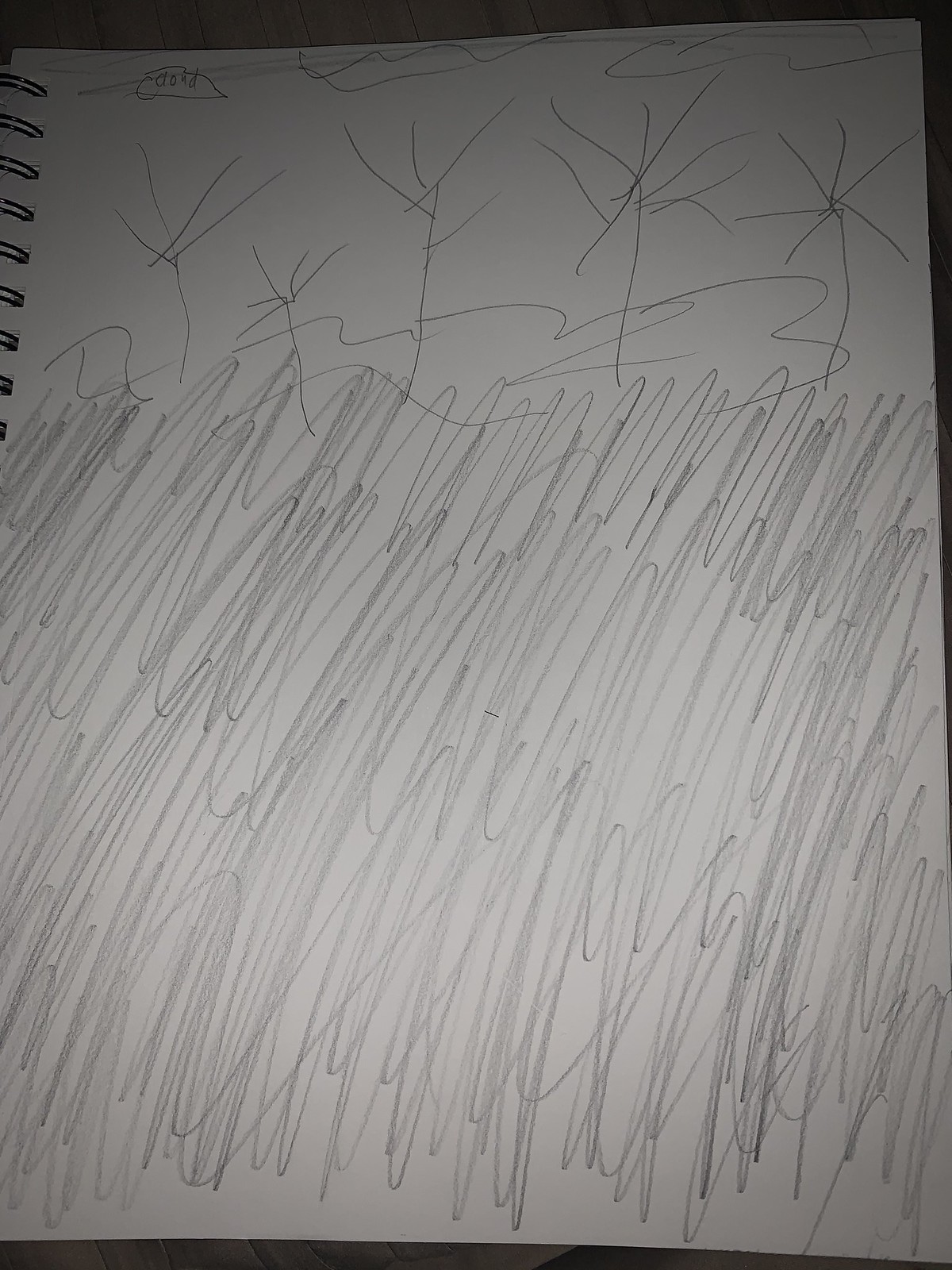This pencil drawing, featured on a page from a spiral-bound notebook with visible spirals on the left side, presents an intricate and somewhat abstract scene. The bottom two-thirds of the page is densely filled with chaotic yet deliberate scribbles, which could be interpreted as tall grass or another form of dense foliage. Rising from this textured base are five vertical elements of varying heights. These elements resemble either bare trees or simplistic representations of structures like windmills, characterized by vertical lines with additional lines radiating from their tops, evoking a sense of ambiguity between natural and mechanical forms. The upper portion of the drawing sparsely depicts the sky, with a lone cloud on the top left that intriguingly resembles a UFO, adding an element of whimsy or surrealism to the scene. Overall, the artwork captures a balance between meticulous detail and open-ended interpretation.